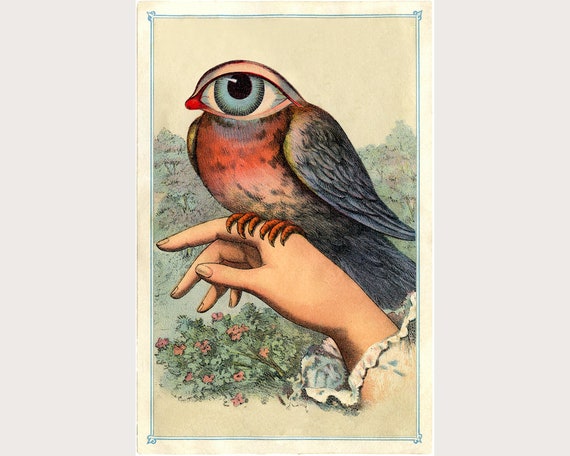This image, reminiscent of a surreal painting or colored pencil illustration, features a close-up of a woman's outstretched hand, which occupies the entire frame. Her sleeve, adorned with a floral pattern and lace frills, delicately accentuates her hand. Perched on her hand is an uncanny bird with a strikingly large human blue eye for a head. The bird's body, detailed with bluish-gray feathers, dark navy and purple wings tinged with yellow at the tips, contrasts sharply with its vibrant red, mottled chest. Orange claws grip the woman's hand, and a tiny orange beak extends seamlessly into the eye, giving the appearance of an eyelid on top of its head. The background is filled with lush, verdant trees and a small flowered bush, adding a naturalistic depth to the seemingly fantastical scene. The entire illustration is set against an off-white poster that has an eggshell-white outer frame, all placed on a white wall.